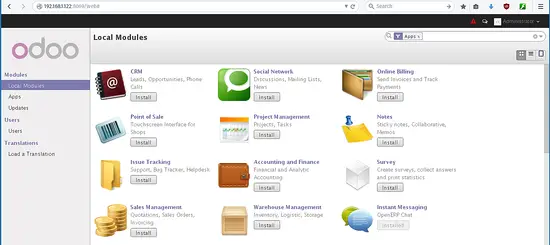Screenshot of the Odoo Site Interface (Local Test Version)

This screenshot captures the user interface of the Odoo site in a local test environment. The logo "ODOO" is prominently featured at the top left, with the first "O" in a lavender purple hue, while the remaining letters "DOO" are in gray. The URL isn't fully legible, suggesting it might be a local development or testing instance of the website.

The interface displays a vertical menu on the left, which includes options such as "Modules," "Local something," "Apps," "Updates," "Users," and "Translations." To the right of this menu, there is a grid layout of various applications, organized in three columns and four rows.

The visible applications include:
1. **CRM** - Icon with an @ symbol on a ring binder.
2. **Social Network** - Icon featuring a speech bubble on a green background.
3. **Online Billing** - Not explicitly described but likely included.
4. **Local Modules** - Indicating offline mode.
5. **Point of Sale** - Icon with a barcode.
6. **Project Management** - Standard project-related icon.
7. **Notes** - Icon showing a Post-it note with a pin.
8. **Issue Tracking** - Standard tracking icon.
9. **Accounting and Finance** - Not explicitly described but likely included.
10. **Survey** - Standard survey icon.
11. **Sales Management** - Standard sales icon.
12. **Warehouse Management** - Not explicitly described but likely included.
13. **Instant Messaging** - Standard messaging icon.

Each application icon is color-coded for easy identification. For example, the "Post-it notes" app has a pin sticking into a Post-it note.

At the top right of the interface, there is a "Search Apps" option, enabling users to search through the applications. The header bar reads "Local Modules." Additionally, a scrollbar on the right side of the screen indicates that more applications are available below the visible area of the screenshot.